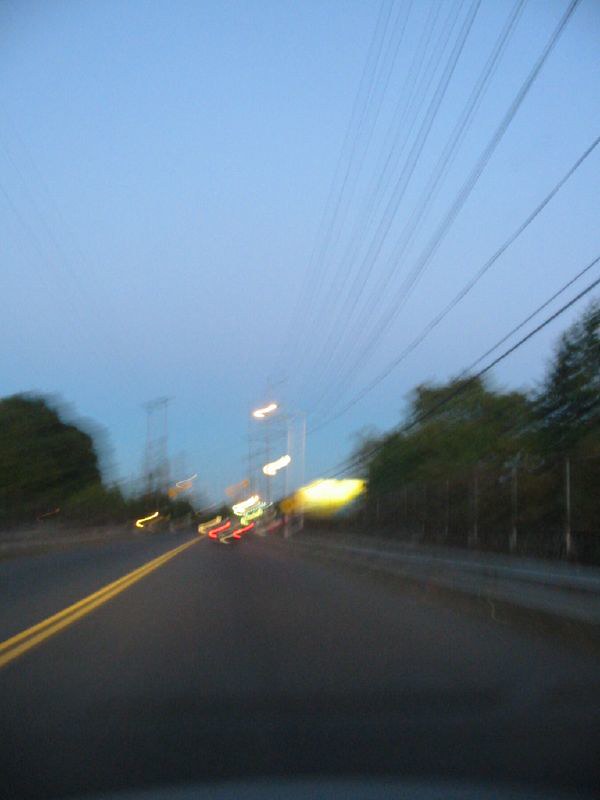A motion-blurred photograph captures a stretch of black asphalt, indicative of a two-lane highway marked by bright yellow lines. The image suggests it was taken from a moving vehicle, as the perspective aligns with a driver's viewpoint, though no part of the vehicle is visible. In the distance, the smear of red brake lights indicates other vehicles ahead. An expansive blue sky frames the scene, suggesting the time is either dawn or dusk due to the soft lighting. To the right, lush green trees border the road, while above, a web of at least ten power lines spans across the sky.